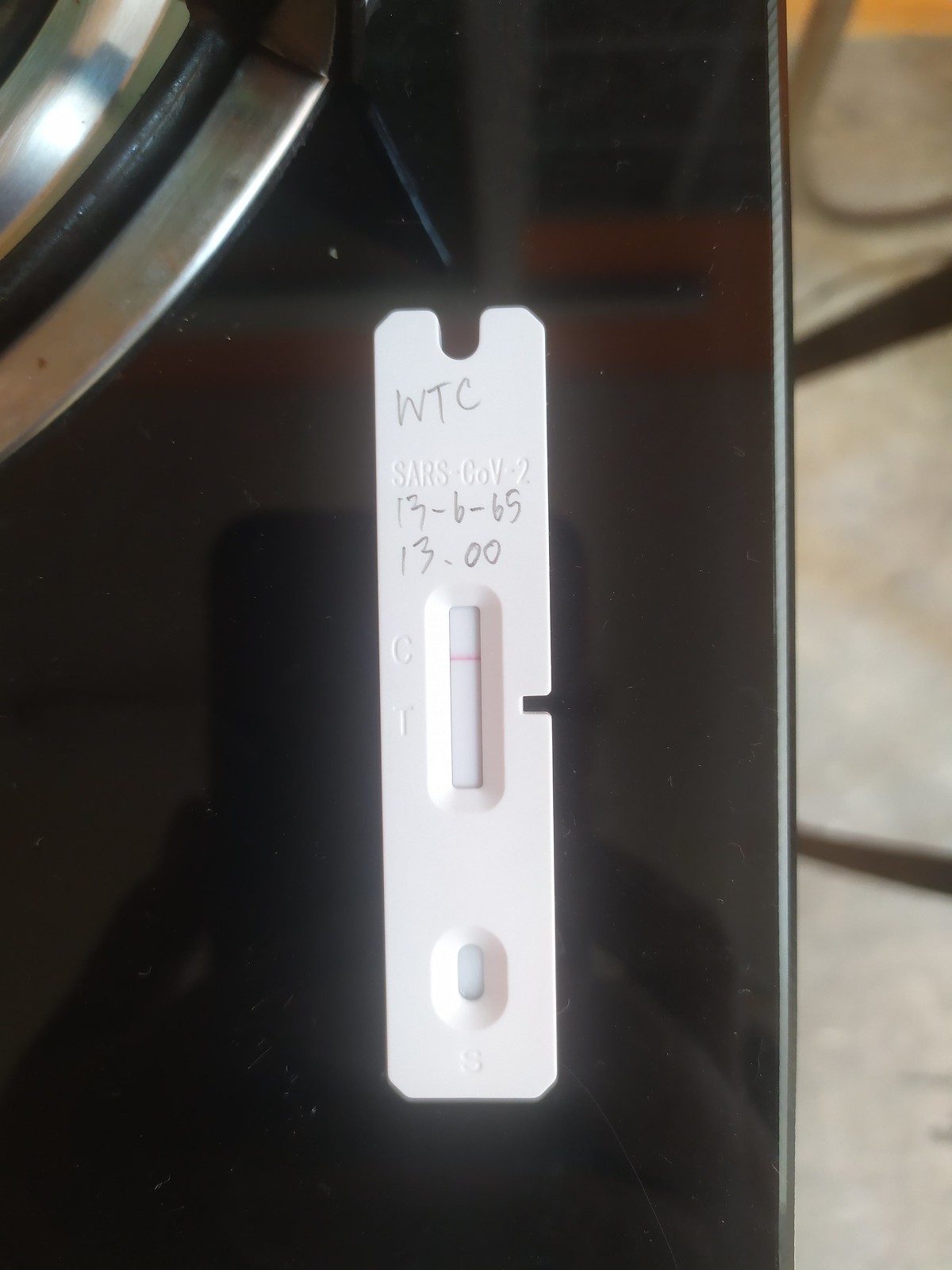The photograph features a close-up of a white test strip prominently positioned in the foreground against a black backdrop. The test strip, potentially a diagnostic tool such as a pregnancy or COVID-19 test, displays a distinct red line. At the top of the strip, the letters "WTC" are visible, followed by the numbers "13, 6, 15," and "13.00." The image is closely cropped around the strip, rendering the surrounding black object indistinguishable. However, some silver, rounded elements appear near the top, potentially resembling parts of a household item like a dryer door. The background reveals a tan-colored concrete floor with several black cords strewn across it. The overall setting and specific purpose of the test strip remain unclear based on the details provided.